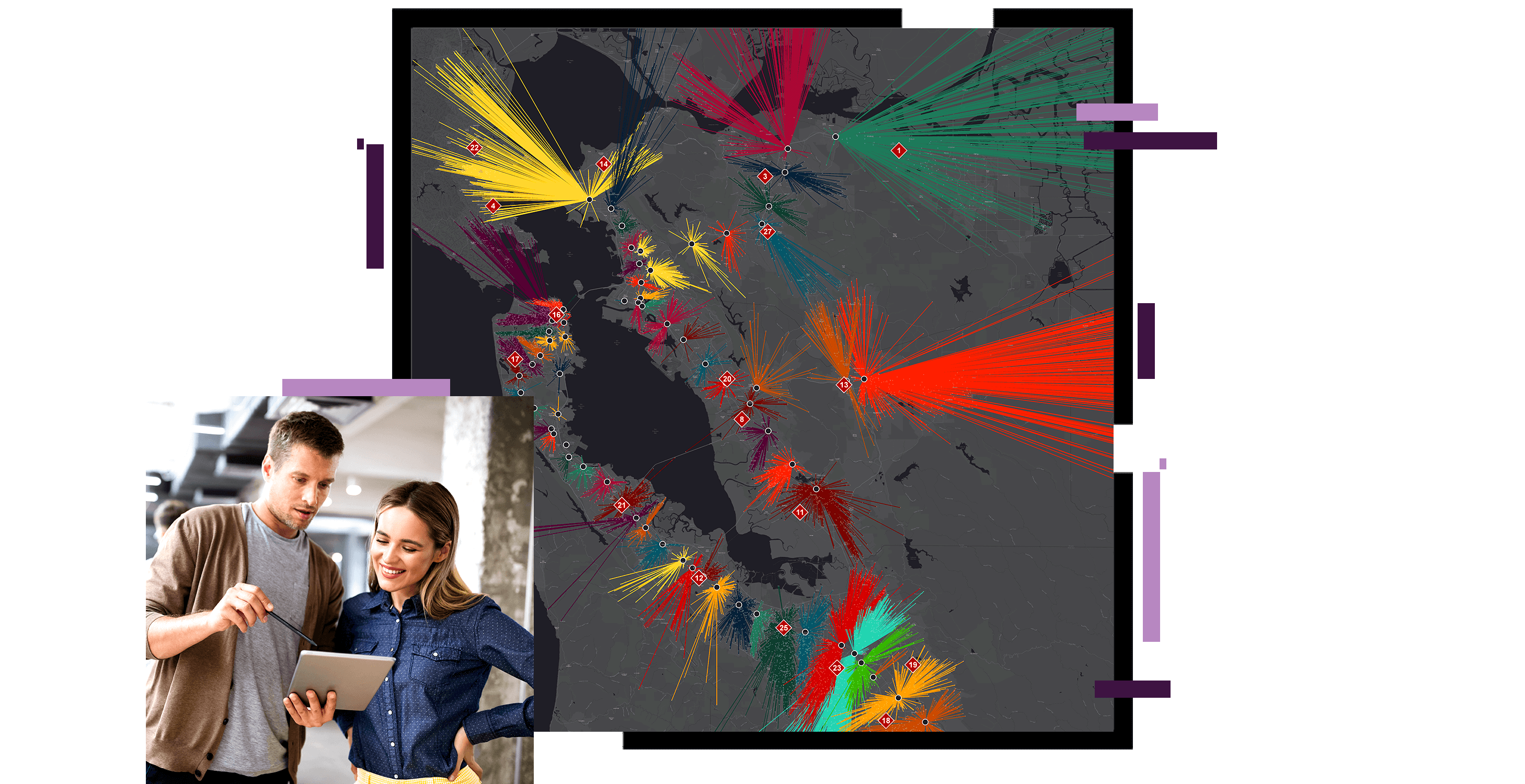This image is a composite of two distinct visuals, artfully blended into one. The primary backdrop features an abstract, colorful painting on a gray background, with splashes of bright colors including reds, greens, yellows, and oranges, reminiscent of vibrant natural patterns or fly-fishing lures. These colors appear to extend like branches or waterways, punctuated by black boxes and dots. Superimposed in the lower corner of this abstract artwork is a smaller, detailed portrait of a man and a woman. The man is engaging the woman by showing her something on a digital tablet, to which she responds with a smile. The scene presents a harmonious juxtaposition, possibly suggesting a connection between digital innovation and artistic creativity.